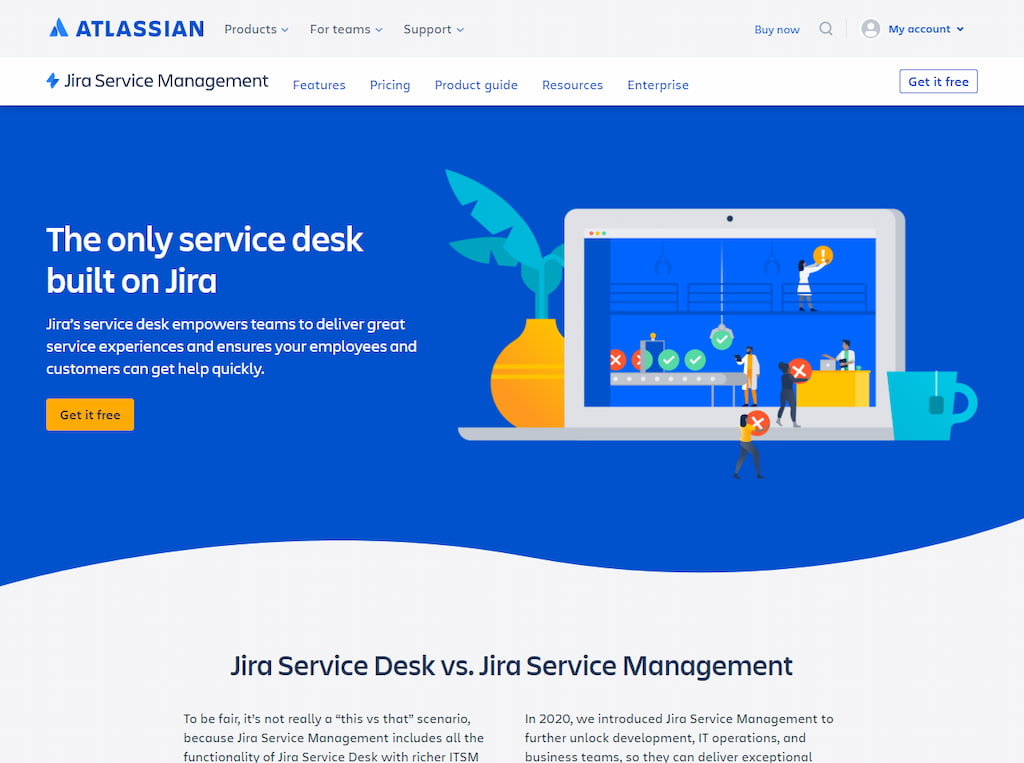**Descriptive Caption:**

This screenshot captures a webpage from a website. At the top, there's a medium gray header. On the left side of this header, a blue logo is visible, featuring a triangle composed of a darker triangle with rounded corners at the bottom left, and a larger trapezoid at the top right. Next to the logo, large blue text in all caps reads "ATLASSIAN" twice. Adjacent to this, in slightly darker medium gray text, are three dropdown options each with a blue caret pointing down: "Products," "For teams," and "Support." 

To the right of these options, there is some negative space followed by blue text reading "Buy now." Continuing to the right, there is a medium gray magnifying glass icon, and next to it, a vertical medium gray separator. Following this, there is a medium gray circle containing a light gray profile picture icon, with blue text beside it reading "My account" accompanied by a blue caret pointing down.

Directly beneath the header, there is a secondary white header. On the left of this header is a slightly squished blue lightning bolt icon. To its right, black text displays "Jira Service Management" (spelled out as "J-I-R-A"). Further right, blue text lists "Features," "Pricing," "Product guide," "Resources," and "Enterprise." 

On the far right of this white header, there is a rectangular white button with a thin blue outline and blue text in the center that says "Get it free."

Below the headers, the main body of the webpage features a background divided into two sections: a blue top portion and a light gray bottom portion. These sections meet in a wave-like seam. In the top left of the blue portion, bold white text reads: "The only service desk built on Jira."